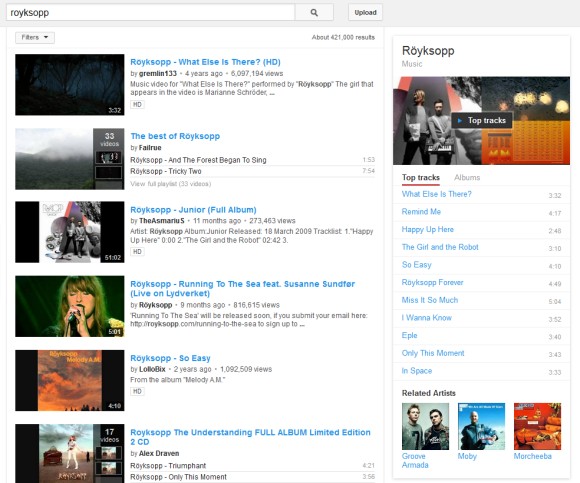A white-background search results page displays a variety of videos related to "Rocky SOP." There is a magnifying glass icon next to the search bar, suggesting the option to refine searches, and an upload button. Filters indicate around 421,000 results are available.

1. The first video listed has a timestamp of 3 minutes and 32 seconds and is titled "Rocky SOP (HD)."
2. The second video is called "The Best of Rocky SOP."
3. The third video, with a duration of 51 minutes and 2 seconds, is labeled "Rocky SOP Jr. (Album)."
4. The fourth video, 5 minutes and 1 second long, is titled "Rocky SOP - Running to the Sea feat. Suzanne Sundfør (Live on Lydverket)."
5. The fifth video, lasting 4 minutes and 10 seconds, is titled "Rocky SOP - So Easy."
6. The sixth video, "Rocky SOP - The Understanding (FULL ALBUM) [LIMITED EDITION 2 CD]," is prominently displayed in all capital letters.

The detailed information includes durations, titles, featured artists, and specific labels such as "HD" or "live on Lydverket."